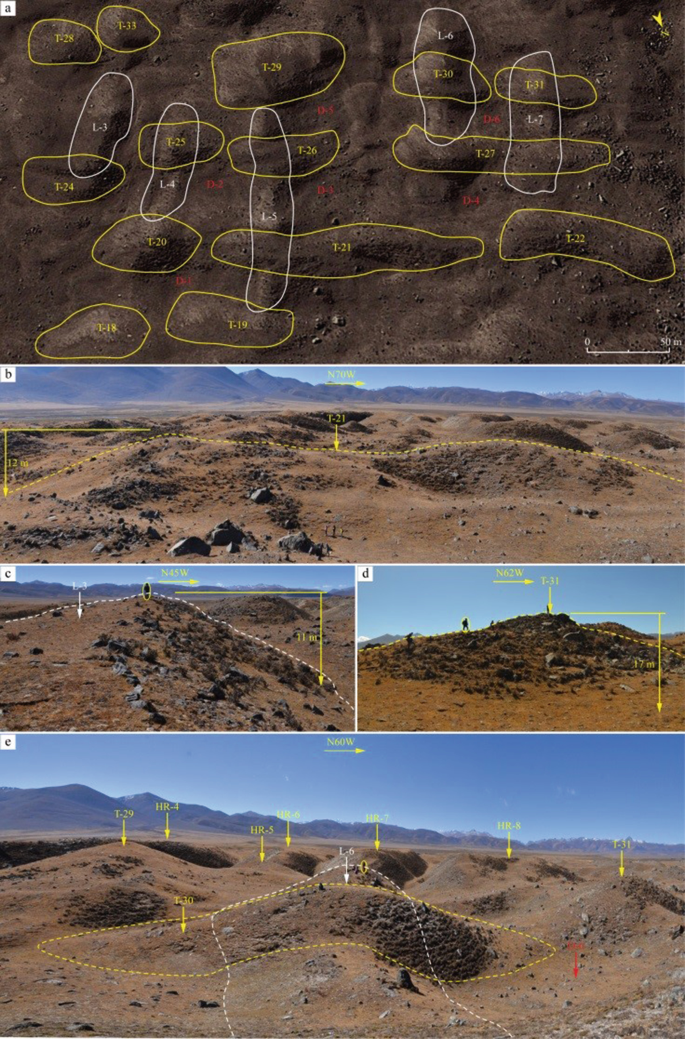The image is a detailed topographical representation of a barren desert landscape, composed of five distinct slides labeled A through E. The area depicted shows a series of raised mounds and hills, with the ground predominantly dark brown and devoid of vegetation. Slide A provides an aerial view, highlighting several mounds with white and yellow circles, each labeled with either an 'L' for vertical mounds or a 'T' for horizontal ones, accompanied by numerical annotations. Slide B offers a side view of the landscape, delineating the contours of the hills with dotted lines and arrows pointing to the highest points. Slides C and D present side perspectives of these elevated areas, including human figures for scale to illustrate the height variations from the lowest to the highest points. The final slide delves into the depth and distance of each mound, creating a comprehensive map that possibly serves strategic purposes, perhaps for navigation or planning in a remote, arid region reminiscent of the Australian outback or Afghan mountains.